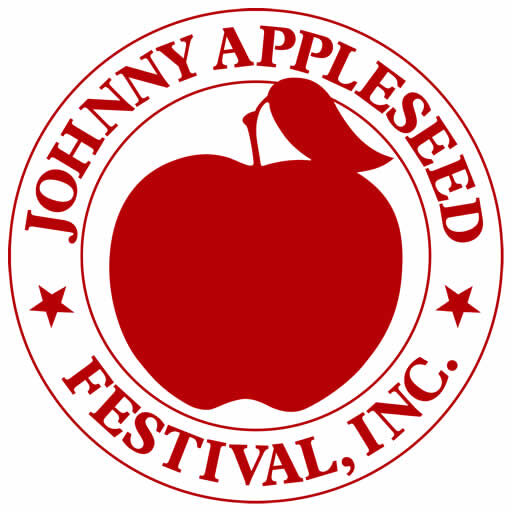This image depicts the logo for the Johnny Appleseed Festival Incorporated. It features a large circular design with an additional smaller circle inside. The entire logo, including the text, is rendered in red and white. The outer circle contains the text "Johnny Appleseed" curved around the top, flanked by two stars on either side. Near the bottom, the text reads "Festival Inc." Inside the smaller circle is a digitally-rendered red apple with a thin stem and a single leaf. The logo is simple yet attractive, characterized by its straightforward block print style and high-quality digital finish, making it easily recognizable.